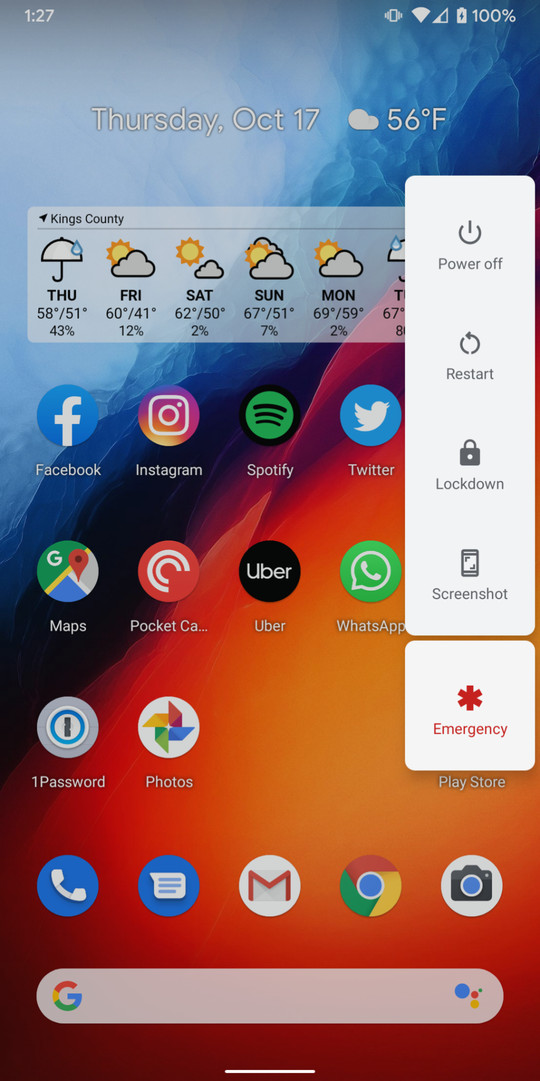The screenshot displays the home screen of a smartphone, capturing various details meticulously. The time is shown at the top left corner as 1:27. Toward the top right, there are several icons indicating phone status: a vibration icon, Wi-Fi with two out of four bars, and a battery meter fully charged at 100%. Below these, the date is October 17th, accompanied by a weather display reading 56°F with a cloud icon.

Prominently featured is a maps application widget spanning a significant portion of the screen. This widget provides a weather forecast from Thursday through Tuesday, with specific details: rain predicted for Thursday, denoted by an umbrella icon, mostly cloudy to partly cloudy conditions for the other days, and rain again forecasted for Tuesday.

Further down, a row of five app icons — Facebook, Instagram, Spotify, Twitter, and Maps — appear slightly skewed. Adjacent to these is a slide-out menu on the right side, presented in white. The menu options include "Power off," "Restart," "Lockdown," "Screenshot," and "Emergency."

Other notable icons include Pocket, Uber, WhatsApp, along with a few that are either obscured or unclear. Toward the very bottom, just above a Google search bar, the screen shows five main app icons: Telephone, Speech Bubble (presumably for messaging), Gmail, Chrome, and Camera.

The background of the screen is a striking graphic depicting a blue ice cave on one side and glowing orange fire rising on the opposite side, meeting at a 45-degree angle, creating a visually dynamic and contrasting image.